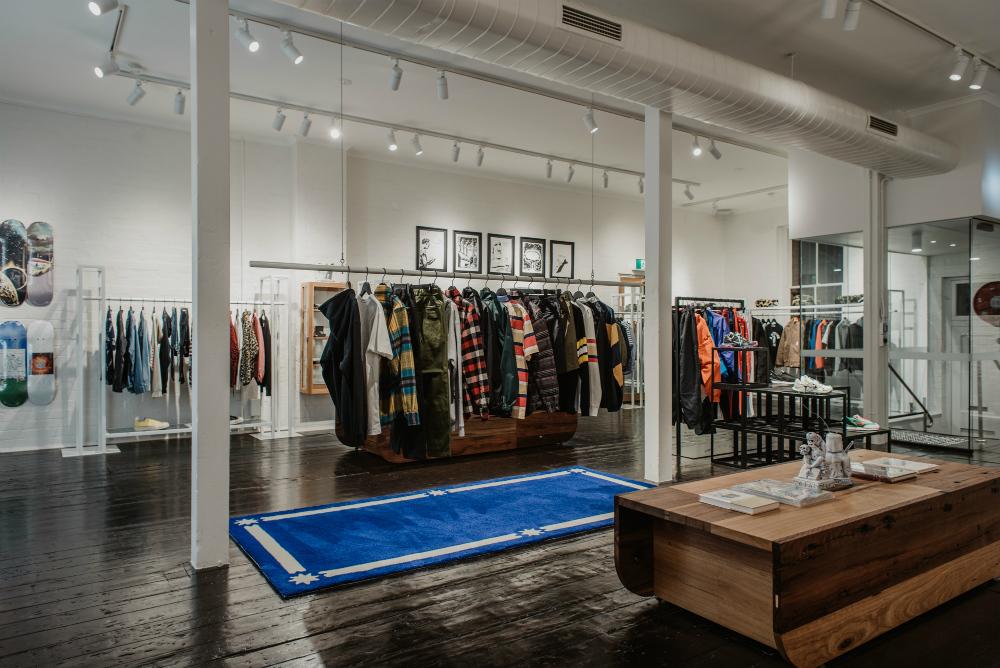The image depicts a spacious and stylish indoor showroom with white walls and dark, glossy hardwood floors. Horizontally arranged bars run across the ceiling, supporting several small light fixtures and air ducts. The room features three cube-shaped beams extending from floor to ceiling. Against the walls and throughout the middle of the showroom floor, various racks display an assortment of shirts and jackets. Five black-framed pictures adorn one of the walls, and there's a distinctive blue rug with a white stripe and star accents at the room's center. A wooden table, located at the bottom right side of the image, holds a few papers. A glass door with a metal railing is situated on the right side, surrounded by high windows that extend approximately ten feet off the ground. Further adding to the uniqueness of the store, there is a notebook, some shoes on display, and intriguing details like the underside of skateboards and a small Dalmatian dog sculpture. The lighting, provided by strategically placed spotlights, and the efficient cooling system, enhance the store's modern and welcoming ambiance.